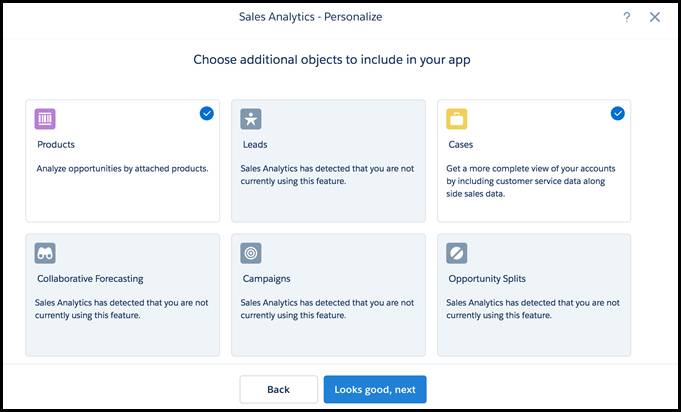This is a detailed screenshot of a personalization settings review screen, likely from a Windows application or website titled "Sales Analytics - Personalize." The screen prompts the user to "Choose additional objects to include in your app." 

Displayed is a grid of six cards, each featuring a unique name, icon, and description. Two of these cards are selected: 

1. **Products** (far left): "Analyze opportunities by attached products."
   - Icon: Colored
   - Background: White
   - Indicator: Blue circled white check mark in the top right corner

2. **Cases** (top right): "Get a more complete view of your accounts by including customer service data alongside sales data."
   - Icon: Colored
   - Background: White
   - Indicator: Blue circled white check mark in the top right corner

The unselected cards include:

- **Leads**
- **Collaborative Forecasting**
- **Campaigns**
- **Opportunity Splits**

These unselected cards appear with dark gray icons on a light gray background, indicating their inactive status.

At the bottom of the screen, there are two navigation buttons: 

- **Back**
- **Looks Good, Next**

These buttons guide the user to continue or review their selections.